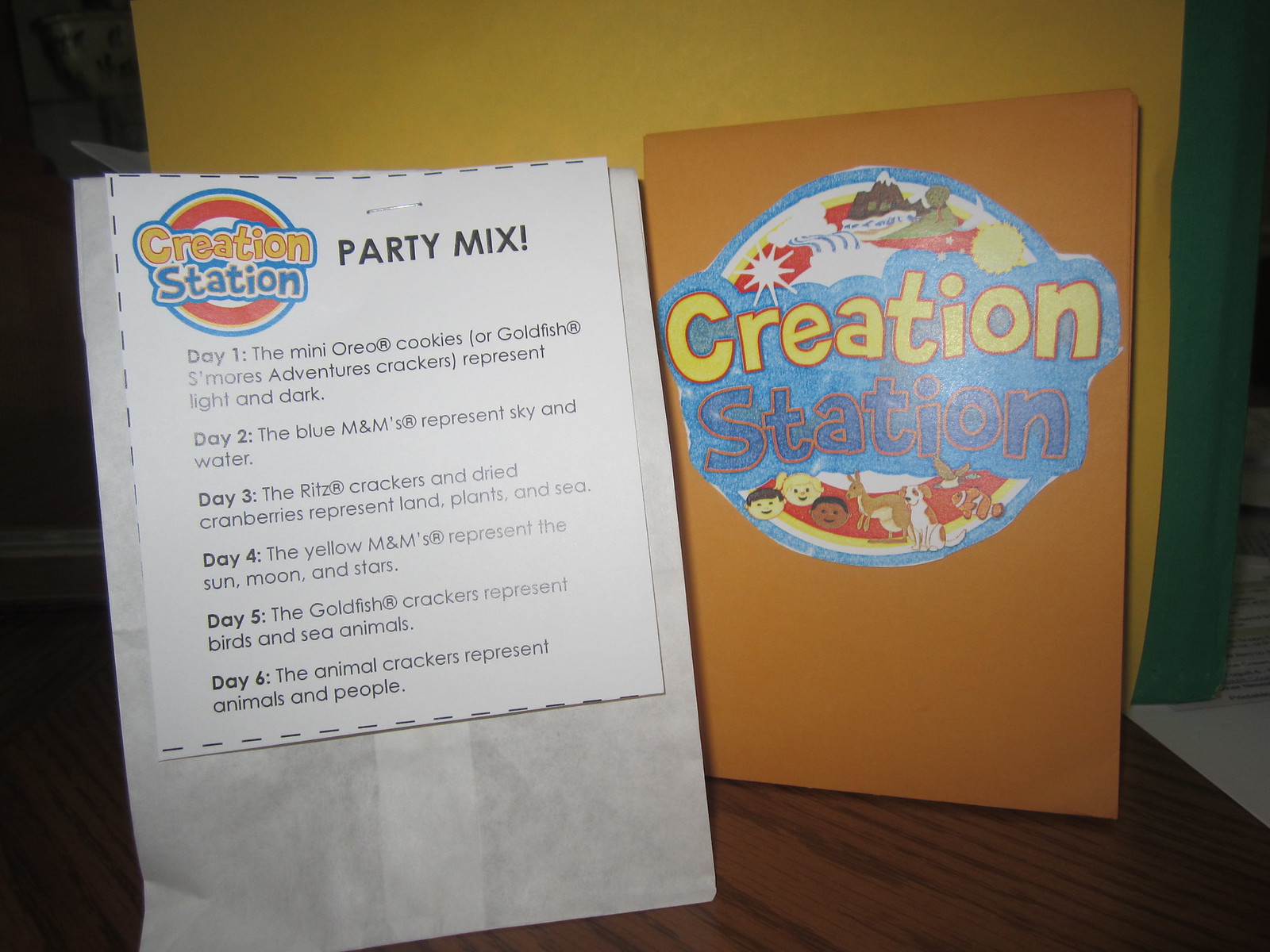The image features a wooden table surface with a white paper bag on the left side. The bag has a piece of white paper stapled to its front with a Creation Station logo prominently displayed in yellow and blue colors, set within a red circle. The paper is titled "Party Mix" in large, black, capitalized letters. Below the title, it outlines a daily snack theme correlating to the days of creation: 

- **Day 1:** Mini Oreo cookies represent light and dark.
- **Day 2:** Blue M&Ms represent sky and water.
- **Day 3:** Ritz crackers and dried cranberries represent land, plants, and sea.
- **Day 4:** Yellow M&Ms represent the sun, moon, and stars.
- **Day 5:** Goldfish crackers represent birds and sea animals.
- **Day 6:** Animal crackers represent animals and people.

To the right of the bag, there is an orange booklet or pamphlet, also labeled with the Creation Station logo. This booklet features more detailed illustrations, including a mountain range, children's faces, a deer, a dog, and Nemo-like fish. Both items are set against a backdrop with a predominantly yellow color that has a green stripe along the edge, creating a vibrant and colorful setup.